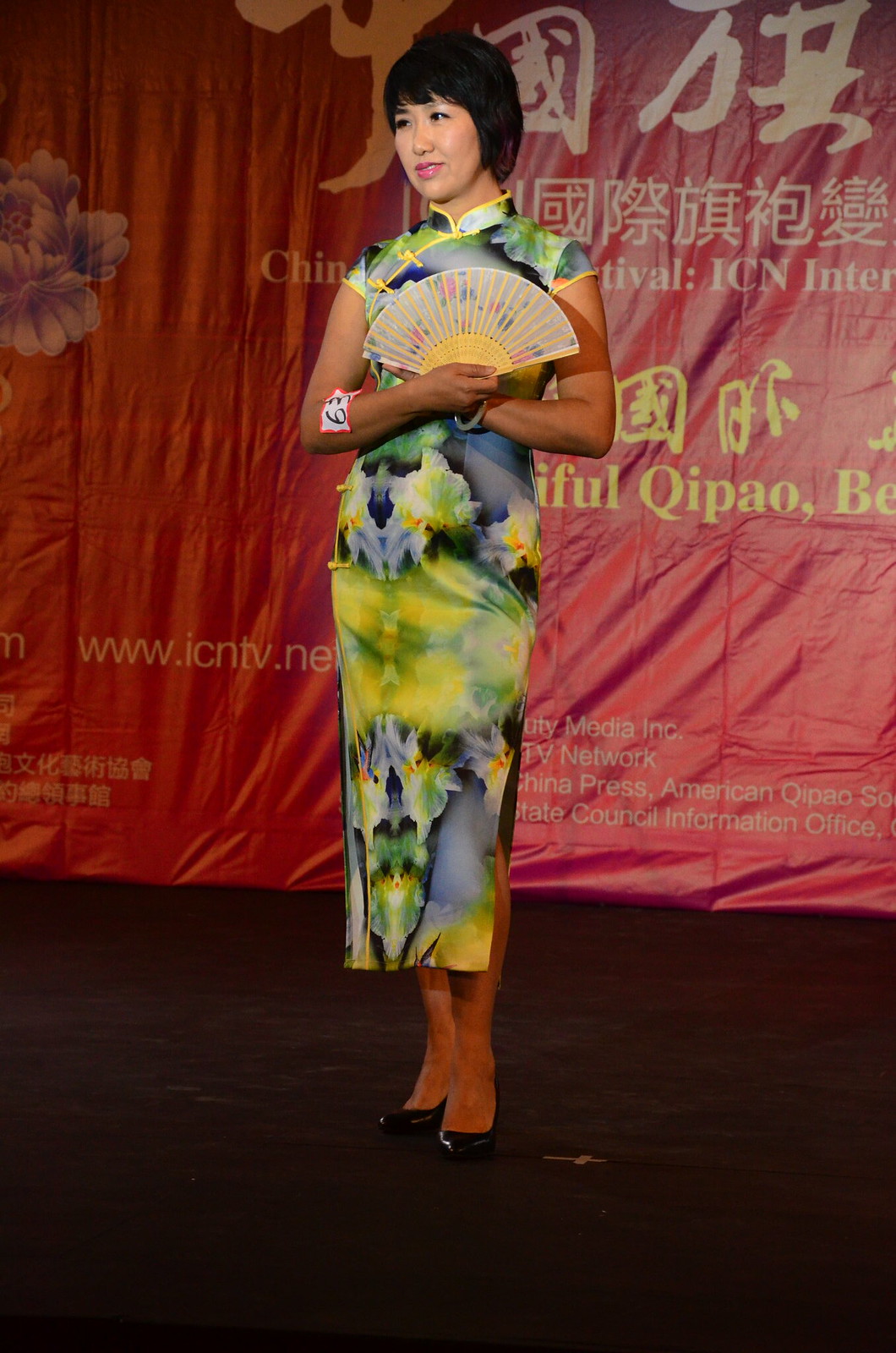The image depicts a striking young Asian woman, likely of Chinese or Japanese descent, standing confidently on a stage. She is adorned in an elegant, traditional floral dress with neon green, yellow, blue, and grey patterns, detailed with yellow edging and piping. The dress features a typical collar, short sleeves just below the shoulder, and a length extending well below her knees, accentuated by a side split. She has short black hair styled in a pageboy cut framing her face, and she complements her look with soft pink lipstick.

Her right forearm bears a sticker with the number 63, possibly indicating her participation in a beauty contest. She stands with her arms folded, holding an open oriental-style fan in front of her chest. 

Behind her is a large reddish fabric banner adorned with a mix of flowers, designs, and text in Chinese characters alongside some English text, including "www.icntv.net." The banner and stage setup suggest a formal event or competition, further emphasized by the black heels she wears. The banner's yellow and white text, along with its intricate design, adds to the backdrop's visual appeal, framing the poised figure of the woman as the centerpiece of this vibrant and culturally rich photograph.